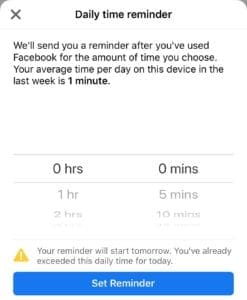The image features a screen capture of a Facebook interface prompting users to set a daily time reminder. At the top, the header reads "Daily Time Reminder" in a clear, bold font. Below the header, the text informs users, "We'll send you a reminder after you've used Facebook for the amount of time you choose." The interface then displays the user's average daily Facebook usage over the past week, highlighting "1 minute" in bold for emphasis.

Proceeding downward, there's a blank white space followed by a faint gray line. The time selector appears next, starting from "0 hours 0 minutes" on the left and right, respectively. As the user scrolls down, increment marks appear: "1 hour 5 minutes," then "2 hours 10 minutes," with the subsequent portion cut off from view.

Further down, a faint gray line separates the current section from a warning message. A yellow triangle containing a white exclamation mark indicates, "Your reminder will start tomorrow. You've already exceeded this daily time for today." 

At the very bottom, a long, skinny rectangular button in blue offers the option to "Set Reminder" in a whitish-tan font, positioned centrally within the button.